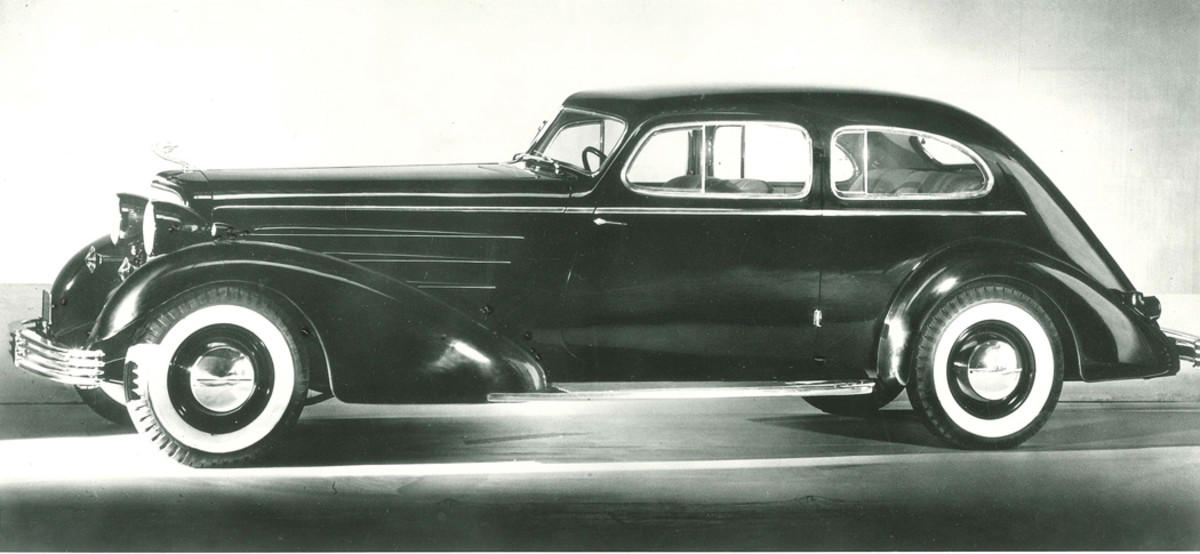This black and white photograph captures an exquisite vintage automobile, likely from the late 1930s or early 1940s. Positioned centrally in what appears to be a showroom, the car exudes an air of timeless elegance. The vehicle boasts a shiny black finish and is characterized by its incredibly long hood, which extends toward the left side of the photo, nearly dominating the length of the car. Chrome accents highlight its sophisticated design, including a gleaming chrome front bumper and three stylish chrome strips adorning the sides of the hood. 

Further enhancing its classic appeal, the car features smooth, flowing fenders that transition gracefully from the engine to the front door, each encapsulating narrow tires with distinctive white walls and gleaming chrome hubcaps. The door handles are positioned on the front side of the two doors, a hallmark of cars from that era, and the doors themselves are designed to open backward with the hinge at the rear. This two-door sedan offers seating for four passengers, with the rear of the vehicle sharply curving downward, leaving little to no trunk space.

Distinctive features include a prominent hood ornament, reminiscent of a Bentley-style figurine, adding to the vehicle's luxurious aura. Overall, this car embodies the transition of early automobiles from utilitarian carriages to symbols of luxury, emphasizing fluid body lines and opulent detail.